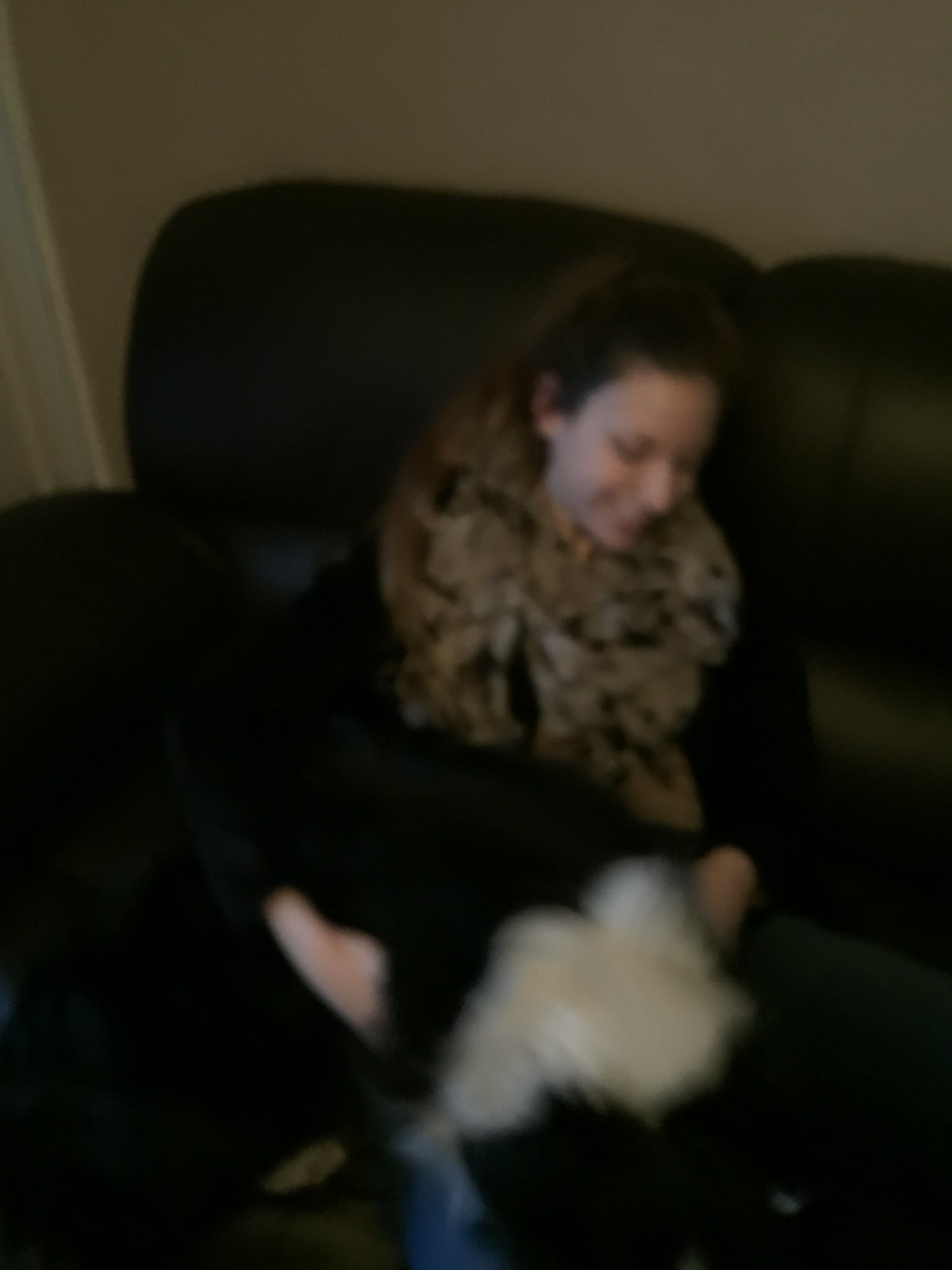The photograph depicts a smiling, light-skinned woman with darker brown hair tied in a ponytail, sitting on a black leather couch indoors. She is dressed in a long-sleeved black top with a large tan and light brown scarf around her neck, featuring a pattern of black spots. The woman is holding a black and white dog in her lap, with her arms wrapped around it as it appears to be either jumping off or onto her. She is leaning slightly to her right. The setting includes a beige or tannish brown wall and white trim running along the corner of the room, with a door frame visible on the left side. The left side of the image is dark and blurry, lacking detail. The overall image is somewhat blurry but captures the warmth and joy of the moment.